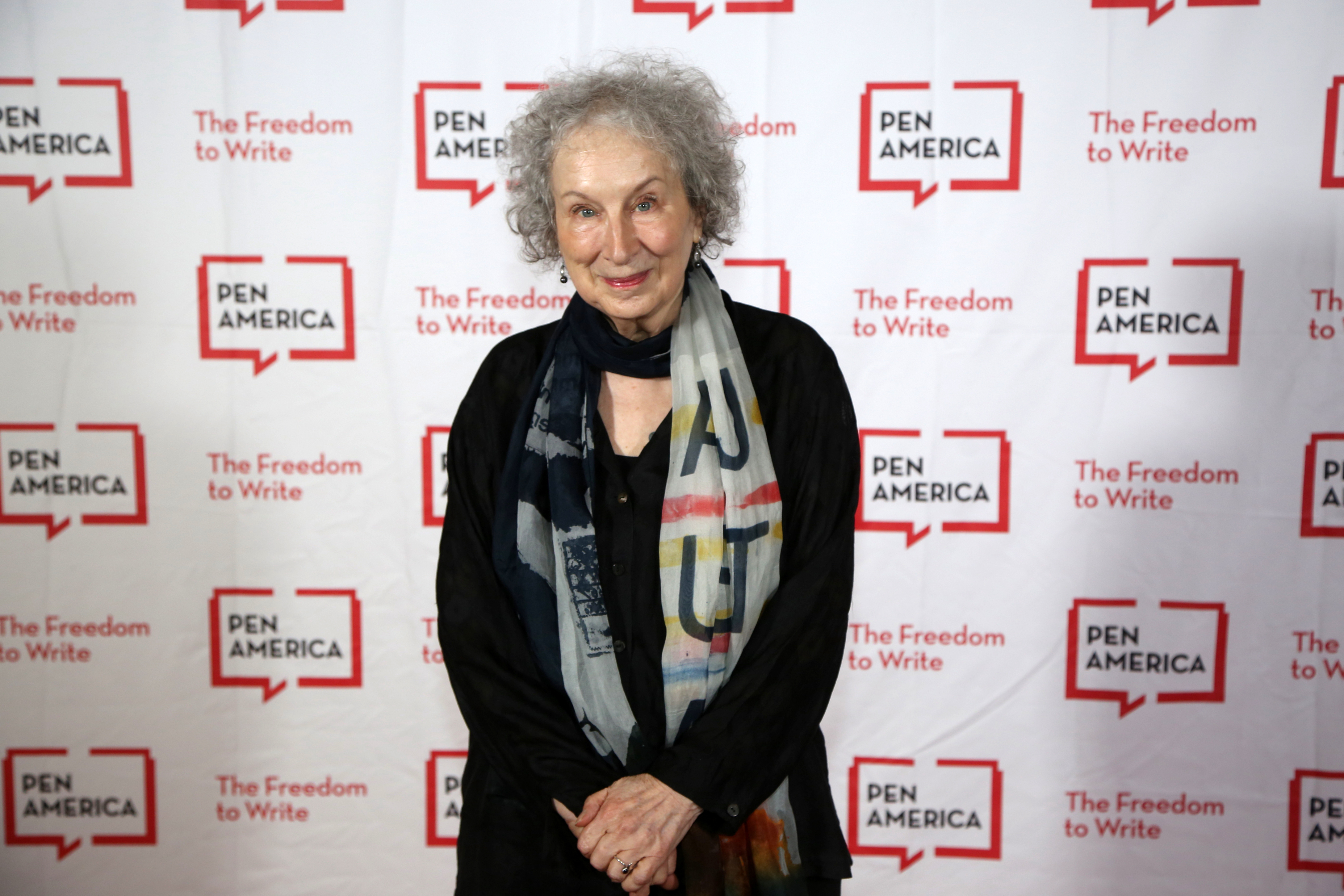In this photograph, an elderly woman, possibly an author, stands prominently in front of a red carpet-style backdrop at a PEN America event. The backdrop features a repeating pattern of the PEN America logo, a black text within a white and red box, alongside the slogan "Freedom to Write" in red text on a white background. The event setting appears to be indoors, with the overall atmosphere suggesting it might be a conference or convention.

The woman is positioned at the center of the image, engaging directly with the camera through her striking blue eyes and a pleasant smile. She has short, curly gray hair and appears to be of Caucasian descent. Her attire includes a long-sleeved black outfit, possibly a button-down shirt, complemented by a colorful scarf. The scarf, draped around her neck, features patterns and lettering that might reference Australia, with the left side showing a gray and black pattern and the right side displaying black letters on a white background interspersed with red, yellow, and blue stripes. Minimal makeup accentuates her natural look, highlighted by a touch of red lipstick and modest earrings.

Her stance is composed yet casual, with both hands gently clasping each other in front of her—a typical pose for such photographical moments. The overall shot encapsulates her dignified presence at a formal literary event, resonating with themes of authorship and freedom of expression.